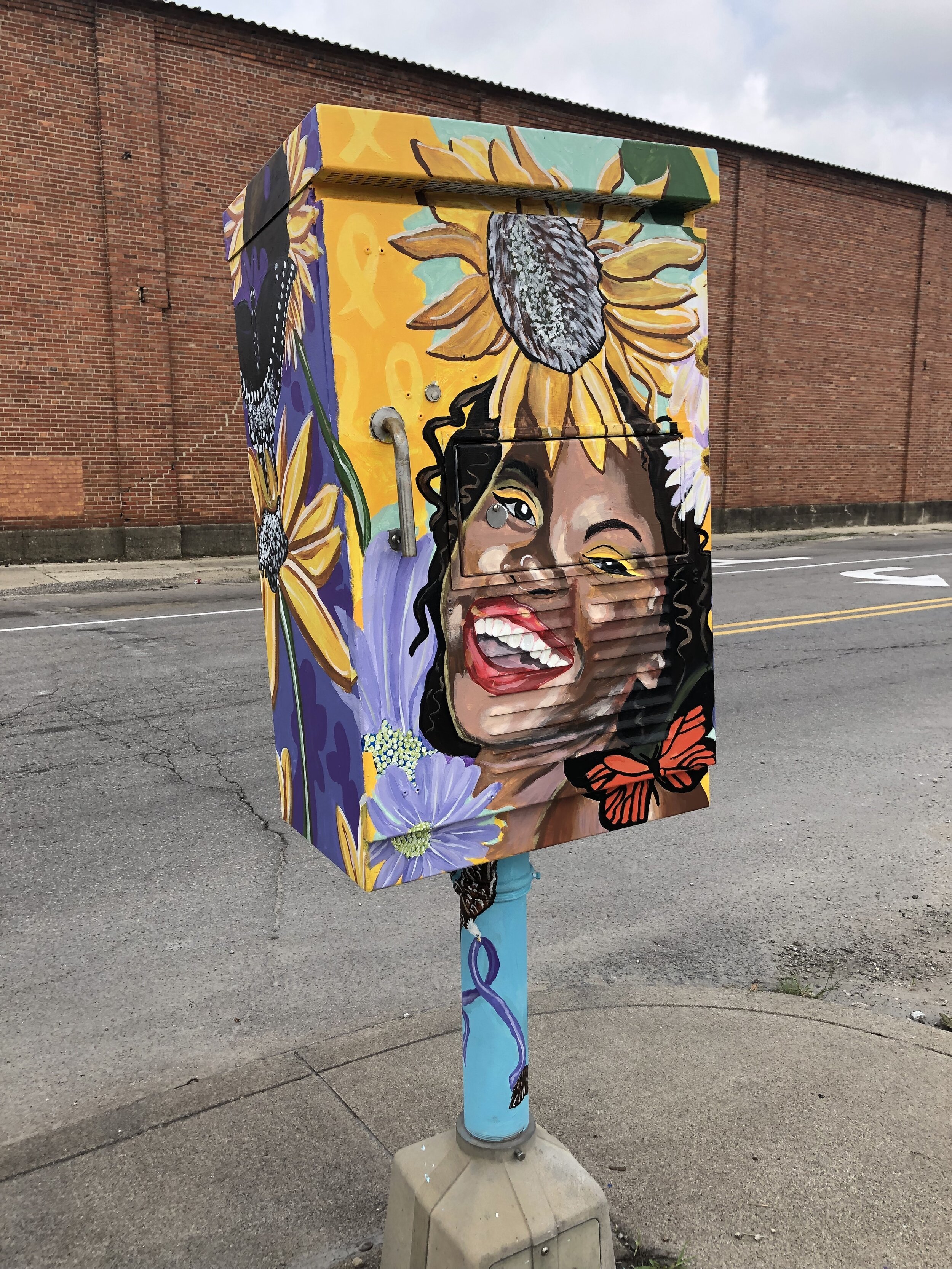The image captures a weathered urban scene featuring a cracked, gray street with yellow traffic lines and a left turn arrow, indicating an old, well-used roadway. The street runs adjacent to a tall, red/brown brick building with a flat, possibly sheet metal roof, spanning the full width of the image. Gray clouds partially obscure the sky above.

In the foreground on the sidewalk, there's a cement-based blue metal pole supporting a rectangular metal box with a handle on its front. The box is adorned with a vibrant mural: a joyful woman with dark skin, black curly hair, a wide smile revealing white teeth, and red lipstick. An orange butterfly rests on her shoulder, while purple flowers frame her face and a daisy floats above her head. The sides of the box are shaded in purple with a large white flower, making it an eye-catching piece of street art.